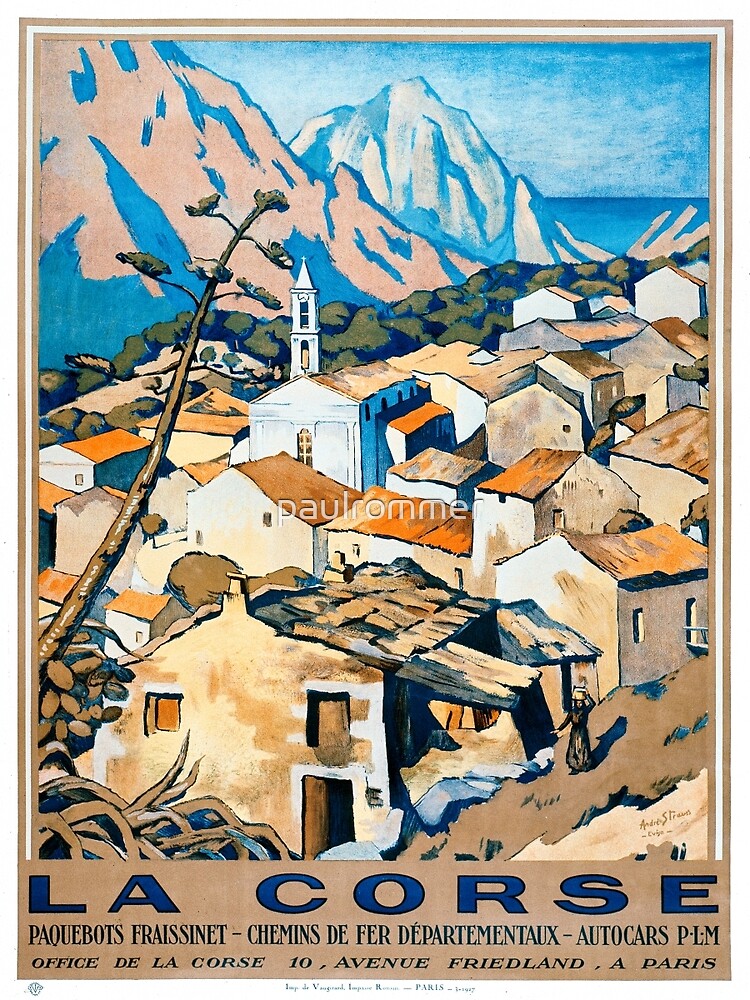This detailed rectangular poster features a picturesque seaside village, depicted in what seems to be watercolor or colored pencil. The scene is viewed from an elevated perspective, showcasing the rooftops of clustered tan and white buildings, accented in blue. A church stands prominently among them, with a tree cascading over the front left of the scene. In the background, majestic mountain ranges rise behind the village, with a river and the expansive blue ocean meeting the vibrant sky on the right.

The artwork is framed with elegant gold, white, and gold borders. Central to the image, in bold white text, are the letters "PAUL ROMER." The bottom border of the poster features a light brown background with several inscriptions in blue letters: “Le Corse, Paquebots, Friesenet, Chemin de fer departmentaux, Auto Cars, PLM, Office de Le Corse, 10 Avenue Freeland, Paris.” A road winds through the very foreground, where a figure can be seen walking, further adding to the charm of the serene village landscape.